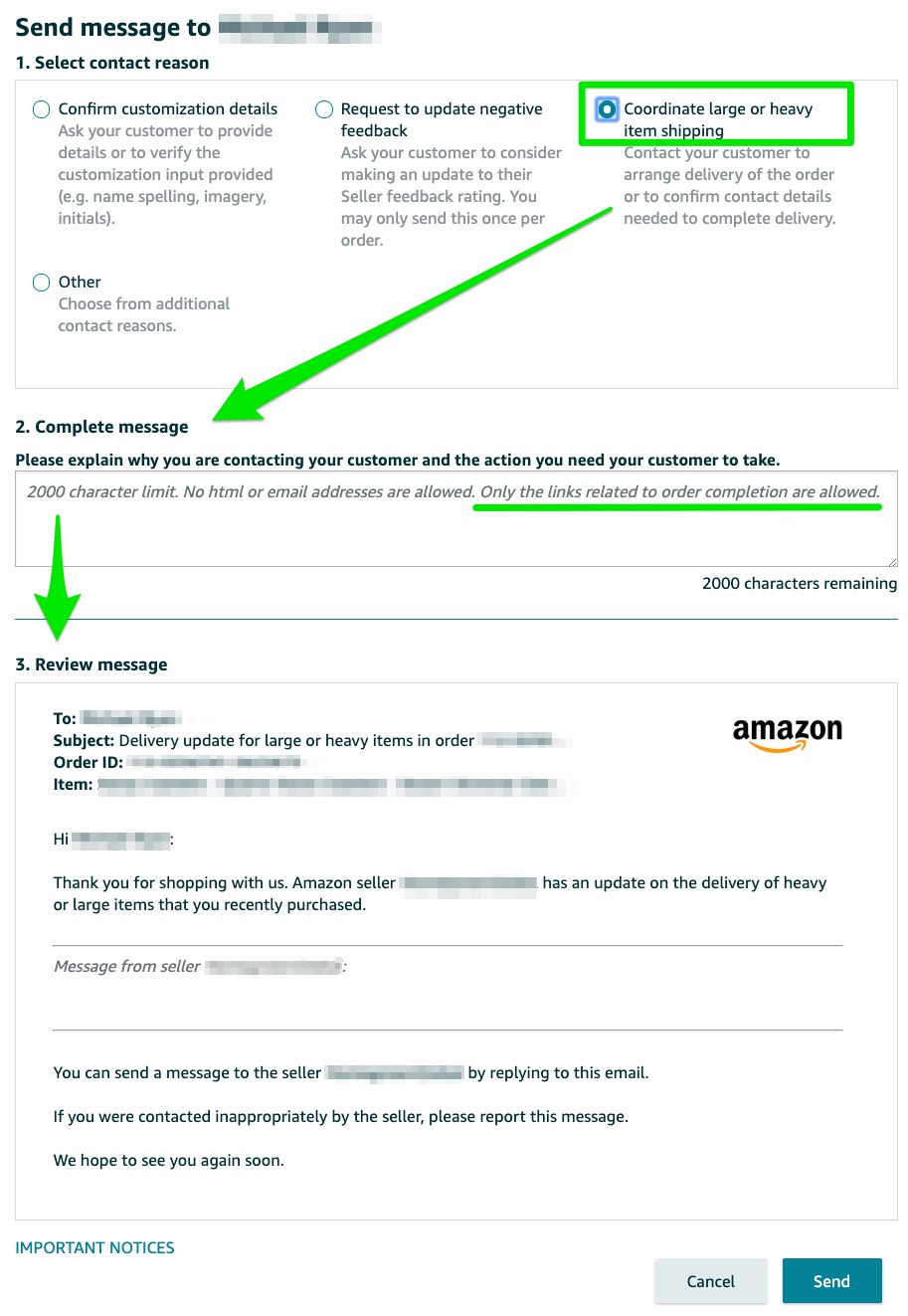**Caption:**

The screenshot shows an instructional webpage designed to guide users through sending a specific type of message on Amazon. At the top, there's a blurred-out section following the prompt "send this message to." Below this, Step 1 asks users to "select contact reasons," offering options such as "confirm customization details," "request update," "negative feedback," and "coordinate large or heavy item shipping," the latter of which is currently selected. 

A green box surrounds this selection, with a green arrow pointing toward a "complete message" section. The form provides instructions to explain the reason for contacting, noting a 2,000-character limit and prohibiting HTML and email addresses but allowing links related to order completion.

Another green arrow points downward to a section titled "Review Message." This part previews the email content, with various fields blurred out for confidentiality, including the subject line "delivery update large heavy items under order," the order ID, and item details. 

On the right side of the preview, an Amazon logo is prominently displayed. The email itself begins with a salutation, "Hi, [Name]," and thanks the recipient for shopping with Amazon. It then mentions an update regarding the delivery of heavy or large items the customer recently purchased. It includes a "message seller" option, instructing users to reply to the email to contact the seller, with a note to report inappropriate contact.

At the bottom, there's a highlighted "Important Notices" link on the left and two buttons on the right: "Cancel" and "Send." This layout appears to be for facilitating streamlined communication related to product descriptions and deliveries on Amazon.